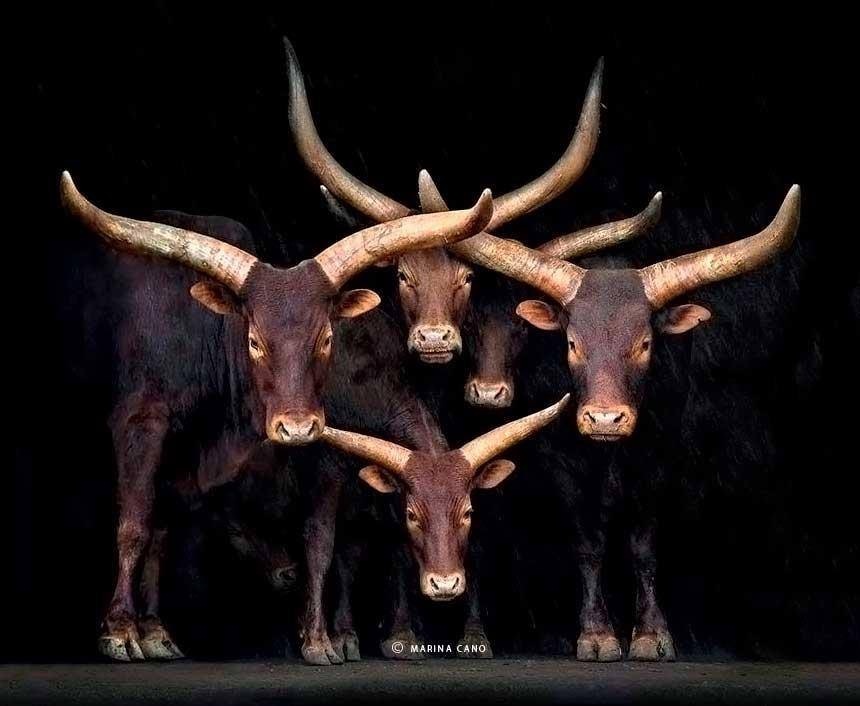In the photograph captured by Marina Cano, five imposing bulls dominate the frame with their direct, piercing gaze. These majestic creatures boast dark brown fur with striking light tan markings encircling their eyes and noses. Each bull is adorned with grand, upward-curving horns that extend from their heads and taper to sharp points, a feature that adds to their formidable presence. Their long ears, matching the tan of their facial highlights, jut out from below the horns, giving them a distinctive, alert appearance. The bulls stand on a black ground that reflects light subtly onto their faces, creating a dramatic effect in the dark setting. Arranged in a staggered formation, two bulls stand on either side, flanking three central figures: one crouched in front, slightly smaller and possibly younger, one just above it, and another looming in the background. The photo exudes a sense of power and unity among these animals, heightened by their synchronized stance and the luminous highlights against the dark backdrop. At the bottom, a discreet white text reads "Marina Cano ©," crediting the artist for this striking image.